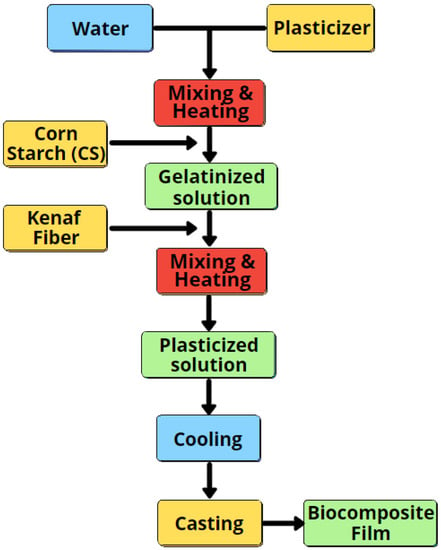This image is a detailed, color-coded flowchart illustrating the process of creating a biocomposite film. The flowchart is structured with various rectangular word bubbles with rounded edges in different colors: blue, yellow, red, and light green. 

At the top, it begins with two primary components: "Water" in a blue box and "Plasticizer" in a yellow box with black writing. A large black arrow points downward from these boxes to a red box labeled "Mixing and Heating." Adjacent to this step, a side arrow highlights the addition of "Cornstarch." 

The next stage, shown in a green box, is "Gelatinization Solution," followed by another arrow pointing to a yellow box indicating the addition of "KNAF Fiber." The process continues with a red box labeled "Mixing and Heating" again, followed by a downward arrow leading to a yellow box labeled "Plasticization Solution." 

Subsequent steps include "Cooling" in a blue box and "Casting" in a yellow box. The final step, positioned to the right side of the chart, is "Biocomposite Film" in a green box.

Overall, the flowchart provides a clear visual representation of the sequential steps and components involved in producing a biocomposite film, from initial mixing and heating to the final product.